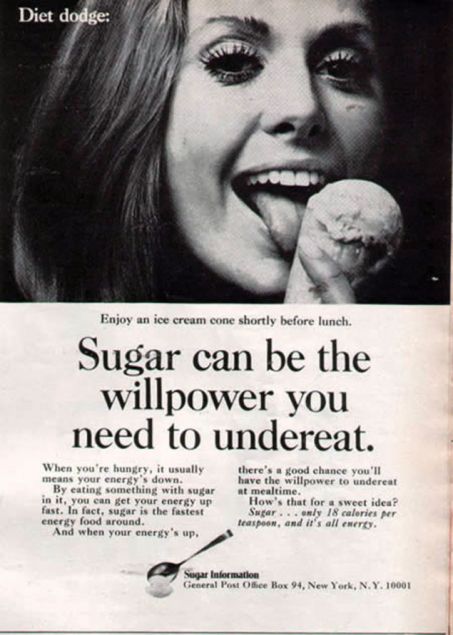The vintage black-and-white advertisement, likely from the 1960s, resembles a magazine page featuring a striking image of a woman with long, dark hair and pronounced eyelashes, smiling as she licks an ice cream cone. The engaging photo captures her white teeth and tongue while she looks directly at the viewer. Prominently placed in the top left corner, the bold white text reads "Diet Dodge." Below the image, a headline asserts, "Sugar can be the willpower you need to under eat," accompanied by the suggestion, "Enjoy an ice cream cone shortly before lunch." The textual content explains that consuming sugar can elevate energy levels, potentially aiding in consuming less food at mealtime, highlighting sugar's role as a fast source of energy. A spoon illustration at the bottom is labeled "sugar information" alongside an address in New York City, noting just 18 calories per teaspoon of sugar. The overall presentation suggests an old advertisement with a focus on sugar's benefits for diet control.